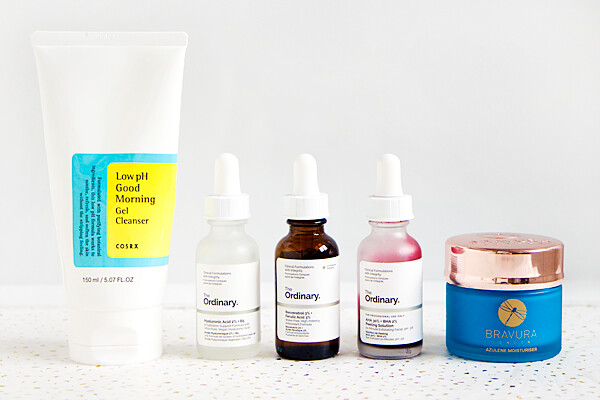This photograph features an array of beauty and cleanser products meticulously arranged on a white counter speckled with black and brown spots. The backdrop is an unadorned white or light gray, allowing the products to stand out. 

**Product Details:**

1. **White Tube:**
   - **Name:** Low pH Good Morning Gel Cleanser
   - **Appearance:** A tall white tube with clear product information displayed on it.

2. **Three Bottles by The Ordinary:**
   - **Appearance:** Each bottle has a white screw top and a distinct label displaying "The Ordinary."
     - **First Bottle:** Contains a clear liquid.
     - **Second Bottle:** Contains a brown liquid.
     - **Third Bottle:** Contains a clear liquid with a red substance mixed inside.

3. **Blue Squat Container:**
   - **Brand:** Bravura
   - **Appearance:** Small, squat, blue container with a large gold screw top.
   - **Design:** Features a picture of a dragonfly inside a golden sun.

The collection of products has been presented systematically, offering a glimpse into a well-curated skincare routine.